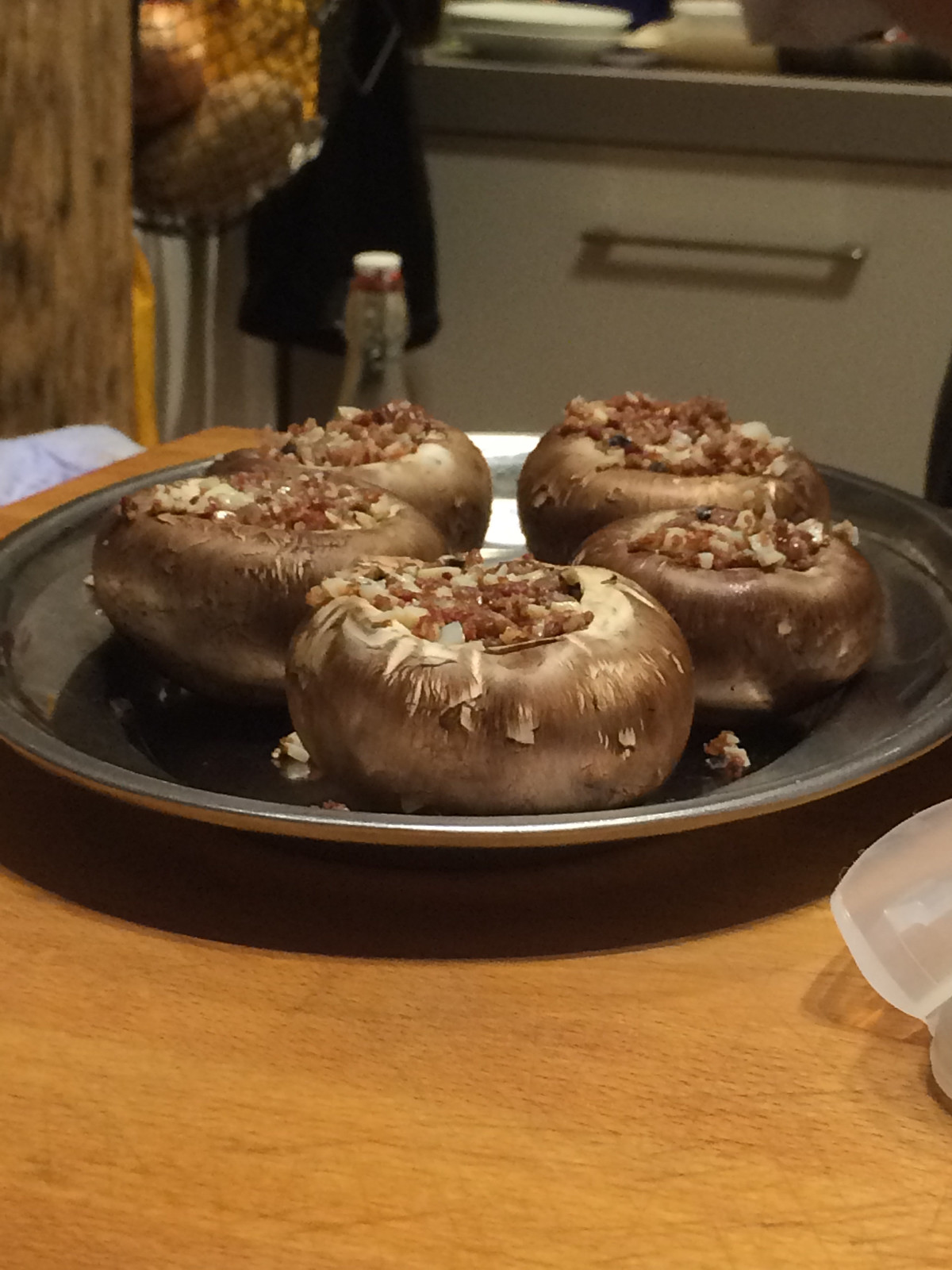The image is a detailed photograph taken in a kitchen. The focus is on a wooden table in the foreground, well illuminated, with a large, round gray platter situated on it. The platter holds five sizable, upside-down mushroom caps, stuffed with a browned, meaty filling interspersed with vegetable pieces, possibly including bacon or a hash-like mixture. The background is dimly lit but contains a distinct gray countertop and a white drawer with a metal handle. A gridded bag is also noticeable in the background. The overall setup suggests a hearty dish likely ready to be served.